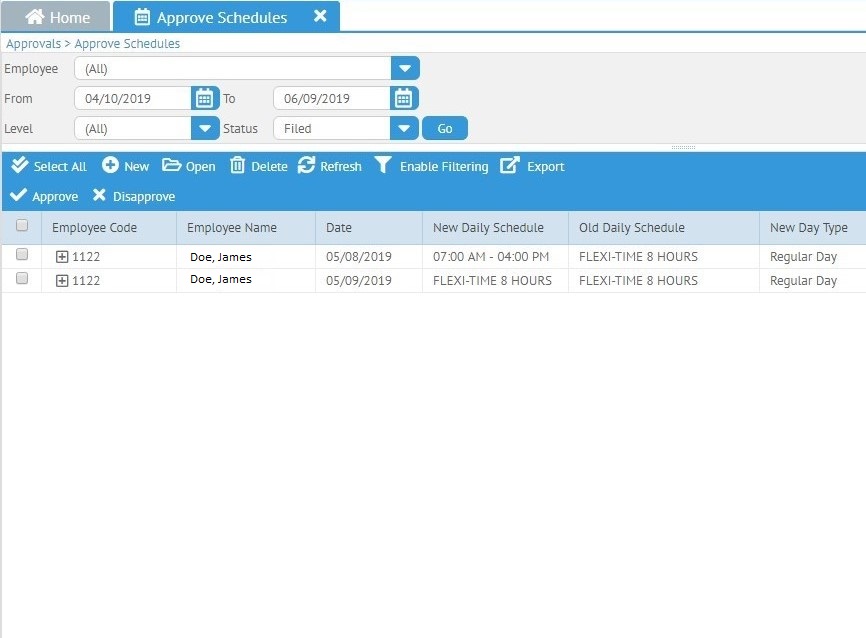In the image, we observe a portion of an application page, focusing on two primary tabs and a detailed section. The backdrop is predominantly white with some black or gray text, interspersed with blue bars and gray sections. At the top, two tabs are visible: a gray "Home" tab with white text, and a blue "Approved Schedules" tab, also with white text.

Beneath these tabs, the layout includes several fields: “Approvals,” “Approved Schedules,” a section for “Employee,” “From” and “To” dates, “Level,” and “Status.” There is a “Go” button to initiate a search or apply filters once the fields are populated.

Directly below this, a blue navigation bar provides options including “Select all,” “New,” “Open,” “Delete,” “Refresh,” “Enable,” “Enable Filtering,” “Export,” “Approve,” and “Disapprove.”

Further down, the page is divided into sections detailing employee-specific information. For example, it lists entries for “Employee Name” such as "Doe, James," accompanied by various dates, employee codes, names, new daily schedules, old daily schedules, and new day types. Each row appears to present comprehensive data for different employees, suggesting it might be a placeholder or a sample dataset.